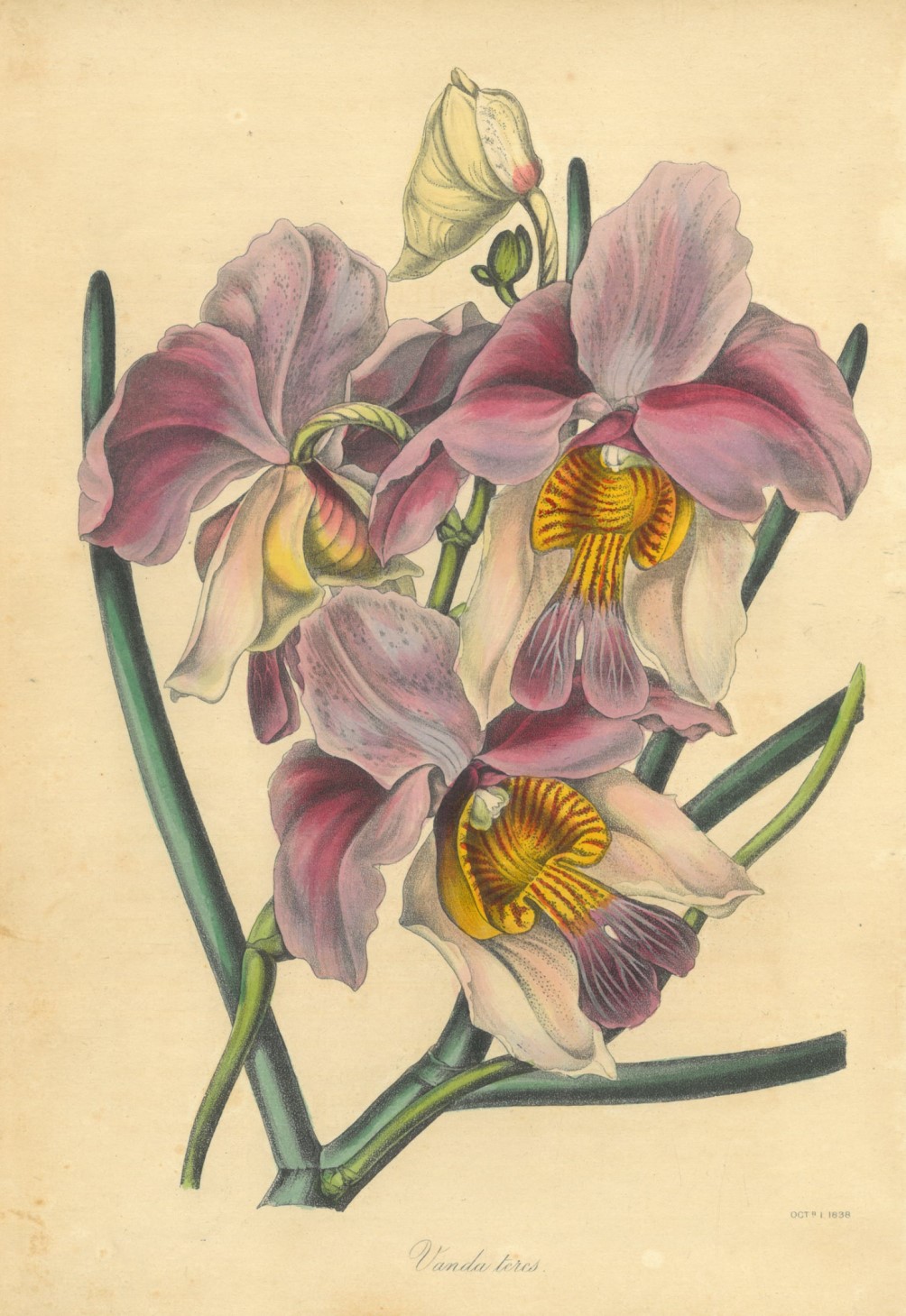This image features a detailed drawing of light pink and light purple flowers, accompanied by green stems and a few small green leaves, all set against a beige background. The flowers also display intricate yellow and red striping on their inner parts. Situated in the lower-right corner is a partially legible date, appearing to read "October 1838." Nearby, a signature, possibly reading "Vonda Perid" or "Vanda Terry," is rendered in cursive, adding an air of authenticity or artistic attribution. The drawing, characterized by its muted and pastel tones, suggests a vintage style reminiscent of greeting cards or seed packets. Some of the flowers are in full bloom, while others show signs of wilting, adding a dynamic, lifelike quality to the portrayal.